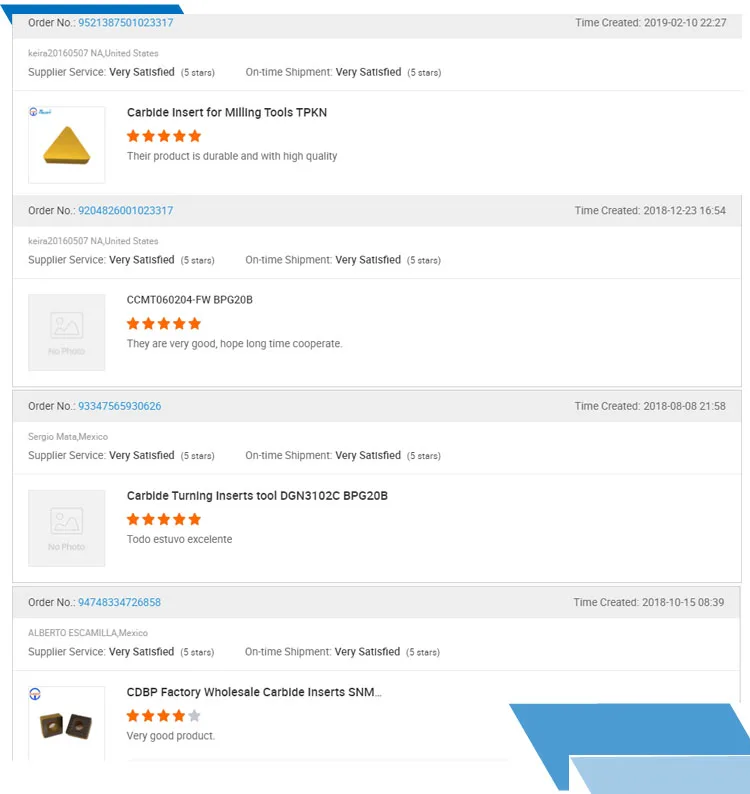The image depicts a screen displaying various supply orders with detailed information. 

At the top left corner, there is **Order Number 9521387501023317**. This information is located in the upper left-hand corner of the first header bar, which is gray in color. In the same bar on the far right, the creation time is shown: **2019-02-10 at 22:27**.

Below these details, it indicates that the order was made by a person in the **United States**. This order is from a **supplier service** that received a rating of "Very Satisfied" with five stars for both on-time shipment and overall service. The ordered product is described as **carbide inserts for mining tools (TPKN)**, which are praised as durable and of high quality. To the left of this section, there is an image of a golden triangle within a square.

The second order displayed is **Order Number 9204826001023317**. The creation time for this order was **2018-12-23 at 14:54**. The item ordered is listed as **CCMT060204-FWB PG20B**, which also received a five-star rating. The review mentions a "Very Good, long-term, long-time cooperation."

The image seems to feature two additional orders following similar patterns, although specific details for these orders are not fully visible in the description.